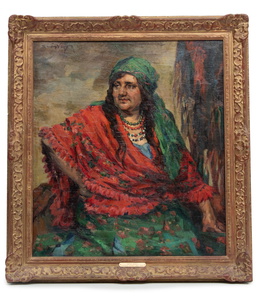This painted portrait depicts a heavyset woman, seemingly from an older era, with an appearance reminiscent of a gypsy. She wears a dark green headscarf and a voluminous red shawl that drapes around her shoulders and down her arms. Her long brown hair cascades to her mid-chest, partially concealed by the headscarf. Adorning her neck are multiple beaded necklaces, featuring green, red, and various other colors. She is dressed in a large green dress, which appears to have red patterns or possibly florets. The woman sits centrally in the frame, slightly turned to her left with a pleasant expression on her face. Her left arm is mostly hidden while her right arm and hand are visible by her side. The backdrop presents a muted, dull sky with green and red hues and scattered dark clouds, adding to the painting's historical ambiance. Encased in a large, tan, ornate frame, the overall aesthetic of the image relies on earthy tones. The painting has no visible signature or title, evoking a sense that it is an old, possibly museum-grade piece, suggestive of a period reminiscent of artists like Rembrandt.